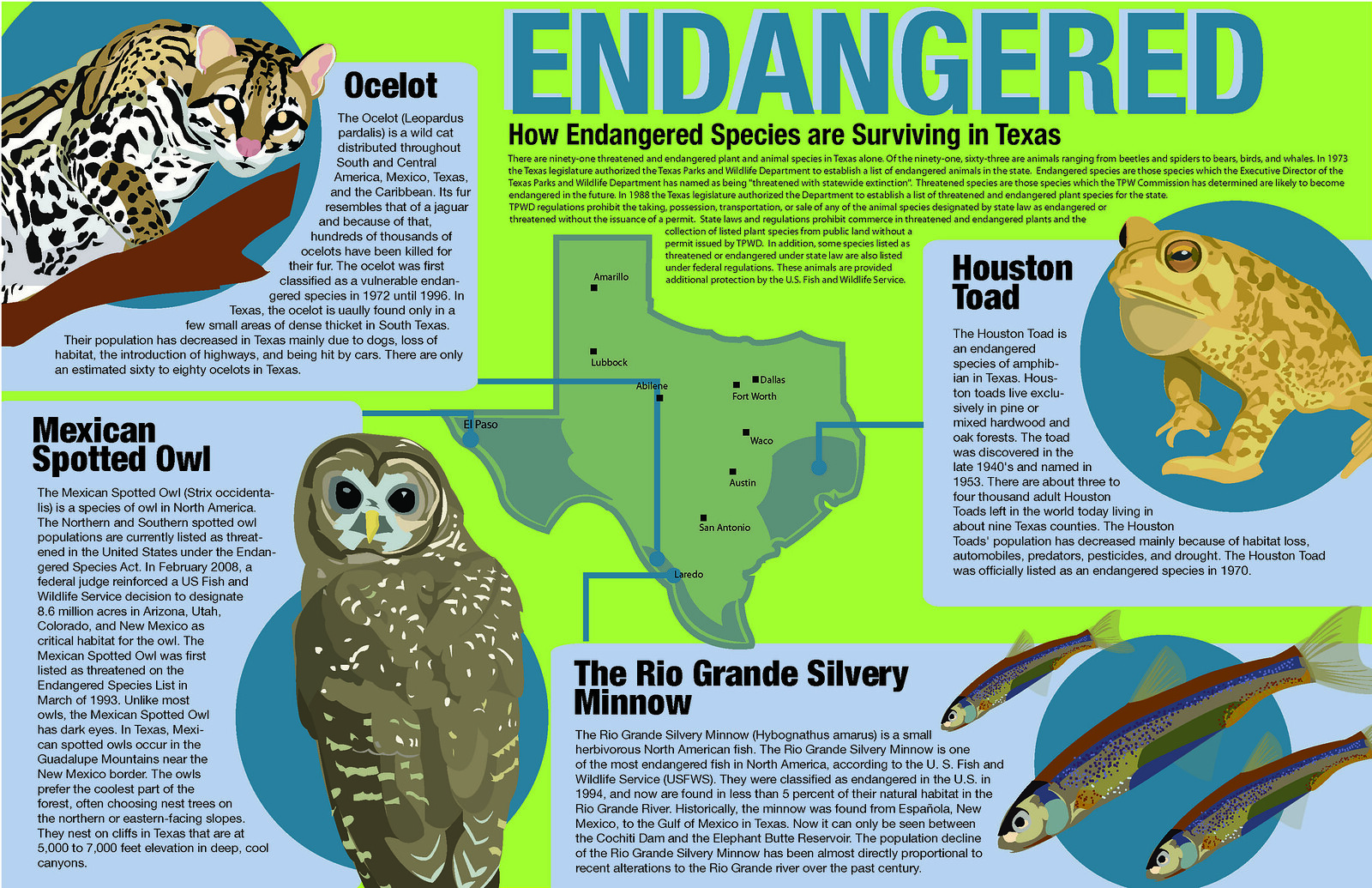The rectangular, neon green informational flyer features the title "ENDANGERED" in large, dark blue capital letters at the very top with a blue border. Directly below, a subtitle in black text reads, "How Endangered Species Are Surviving in Texas," followed by a small, illegible paragraph. The center of the flyer showcases a map of Texas marked with various cities, each connected by blue lines to rectangles around the map that highlight different endangered species in the state. These species include the Ocelot positioned in the top left, the Mexican Spotted Owl in the bottom left, the Rio Grande Silvery Minnow in the bottom right near Laredo, and the Houston Toad to the east of Austin. Each animal is depicted with drawn illustrations and accompanied by descriptive text.